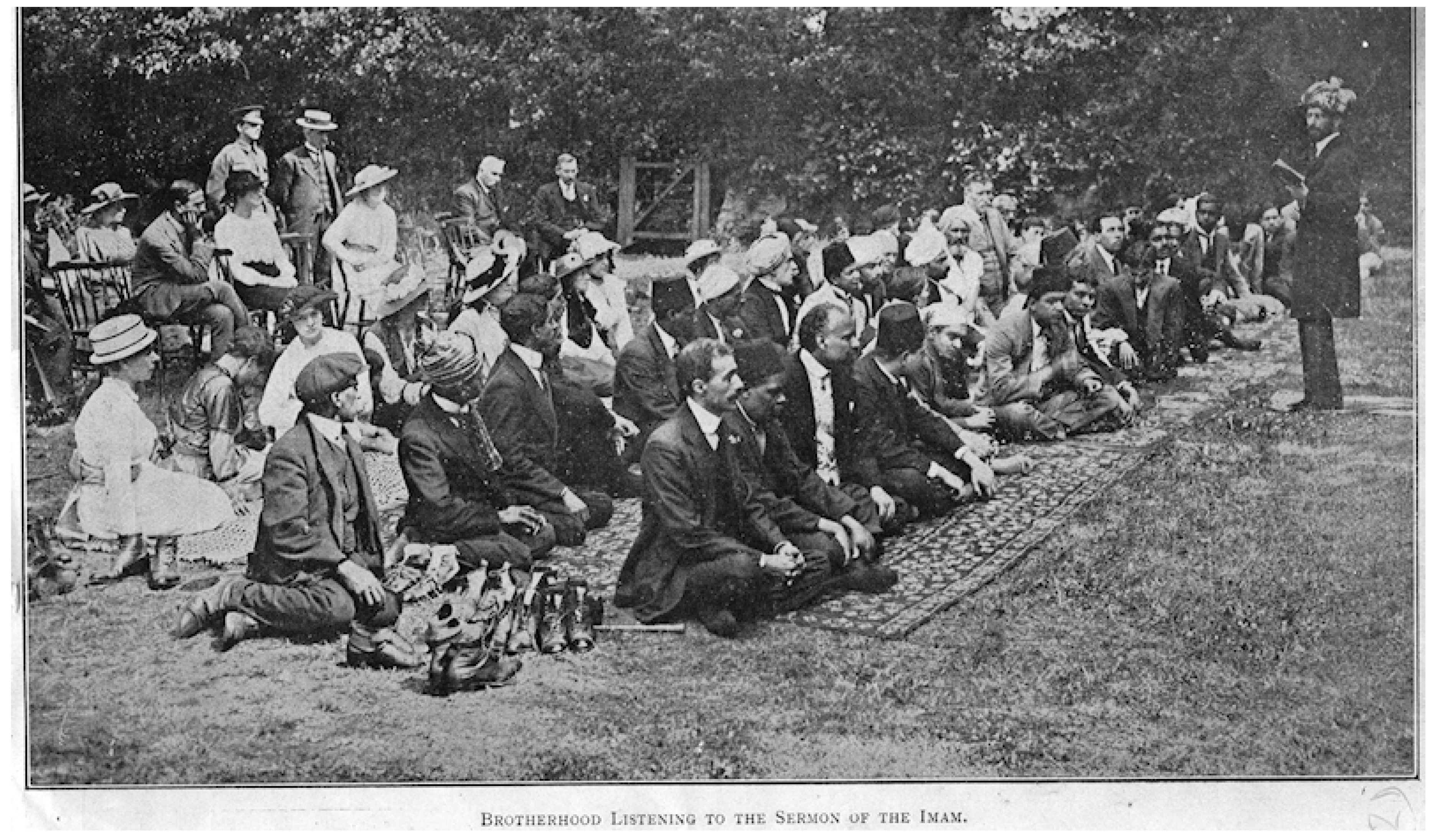The photograph is an old black-and-white image, likely from the early 20th century, showcasing a religious gathering. It captures a man, presumably the Imam, standing on a grassy area, dressed in a formal suit and a headdress, possibly adorned with feathers, holding a book and delivering a sermon. The attentive audience is seated on an ornate floral rug laid out on the grass. The men in the front rows are mostly in suits, some wearing top hats or turbans, while women, dressed predominantly in white dresses and sun hats, are seated further back. In the background, trees can be seen, adding a natural backdrop to this serene scene. The caption below the photo reads, "Brotherhood listening to the sermon of Imam," and the attire and setting suggest that the individuals might be from regions like India or Pakistan. An officer or soldier is also visible among the crowd, suggesting a diverse gathering in terms of roles and attire.